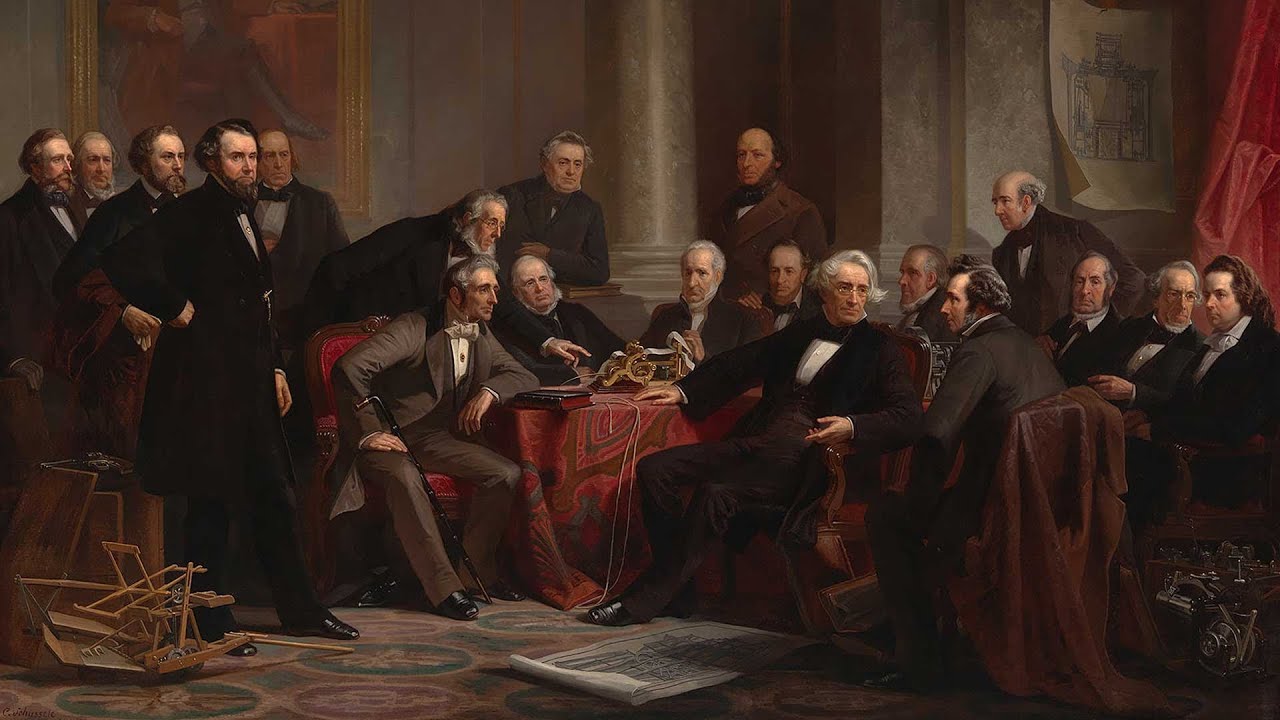The image is a detailed painting, possibly an oil painting, depicting 18 men gathered in an elegant room. They are dressed in 1800s-style suits, and most of them have beards. The setting includes a red carpet with green and red circular patterns on the floor, and they are engaged around a table draped with a red tablecloth. On the table appears to be a telegraph device, which the men seem to be discussing or examining; some are sitting and others are standing, gesturing and pointing towards the telegraph.

To the left, a wooden and metal contraption is visible, while on the right side, another metal apparatus can be seen. The background features a marble column and a large wall painting. In the upper right corner, a hand-drawn blueprint or picture is tacked to the wall beside a red curtain. The composition suggests a scene of intellectual discourse, perhaps focusing on a new invention or scientific plan.